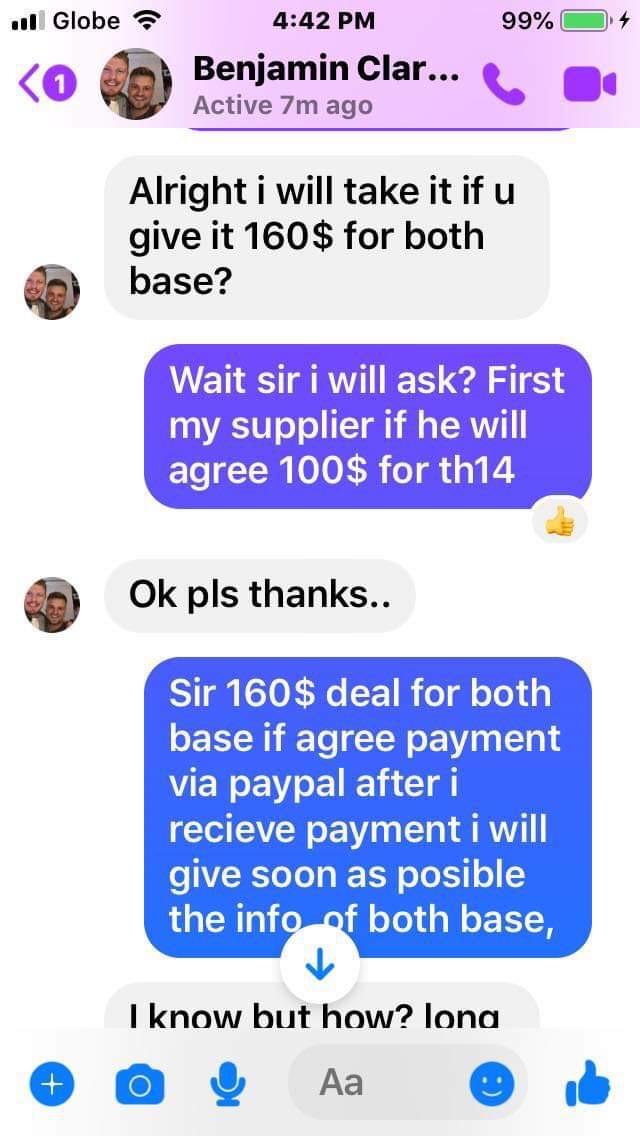The image is a detailed screenshot of a Facebook Messenger conversation, taken on an iPhone. The top of the screen displays standard phone information: full service bars, the carrier "Globe," a Wi-Fi symbol, the time "4:42 PM," 99% battery life with a green battery icon, and a charging symbol. The conversation is between two people, with "Benjamin Klar" being one of them, marked as "active 7 minutes ago." Next to Benjamin's name are call and video call buttons. The conversation unfolds with the first person agreeing to take an item if offered for $160 for both bases. The other person responds by saying they need to check with their supplier if $100 for "TH14" is acceptable, followed by a thumbs-up emoji. The initial person then acknowledges with "ok please thanks." Eventually, the supplier agrees to a $160 deal for both bases, and the final text confirms that payment will be via PayPal and details will be provided after payment. The messages are displayed in alternating text bubbles of different colors, typical of a chat app interface. The visible colors include purple, white, black, green, pink, gray, and blue. The screenshot takes up the entirety of the image, highlighting the text conversation and phone status details.